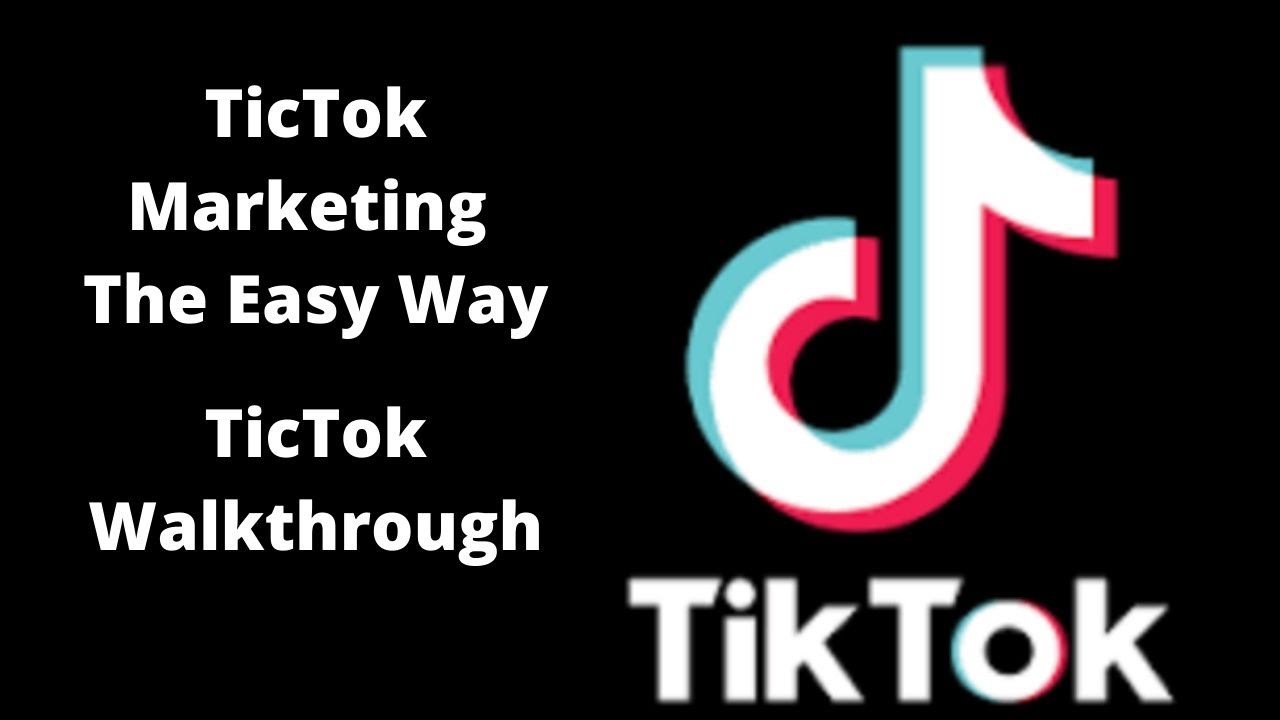This image features a solid black background with contrasting white text on the left side. The text is organized in five lines, each line presenting distinct parts of the title and subheading relevant to the content. The text reads as follows:

1. Tick Tock
2. Marketing
3. The Easy Way
4. Tick Tock
5. Walkthrough

Note that "Tick Tock" is spelled out as "T-I-C-T-O-K", a potential error or a stylized variation.

On the right side of the image, there is a large representation of the TikTok logo. The logo resembles a musical note or a stylized 'D' with a curved downward slope at the top, divided into two colors: teal on the left and pink on the right. These colors blend into the white outline of the logo, creating a striking visual contrast against the black background.

At the bottom right corner of the image, the brand name "TikTok" (spelled correctly as T-I-K-T-O-K with both 'T's capitalized) is displayed. The letter "O" in "TikTok" carries a slight hue of teal on its left side and pink on its right side, complementing the colors within the logo above it.

Overall, this image appears to be a self-made advertisement promoting an easy guide to TikTok marketing, featuring a walkthrough. The combination of detailed text and the prominent TikTok logo creates a clear and visually engaging message aimed at drawing attention to TikTok marketing strategies.